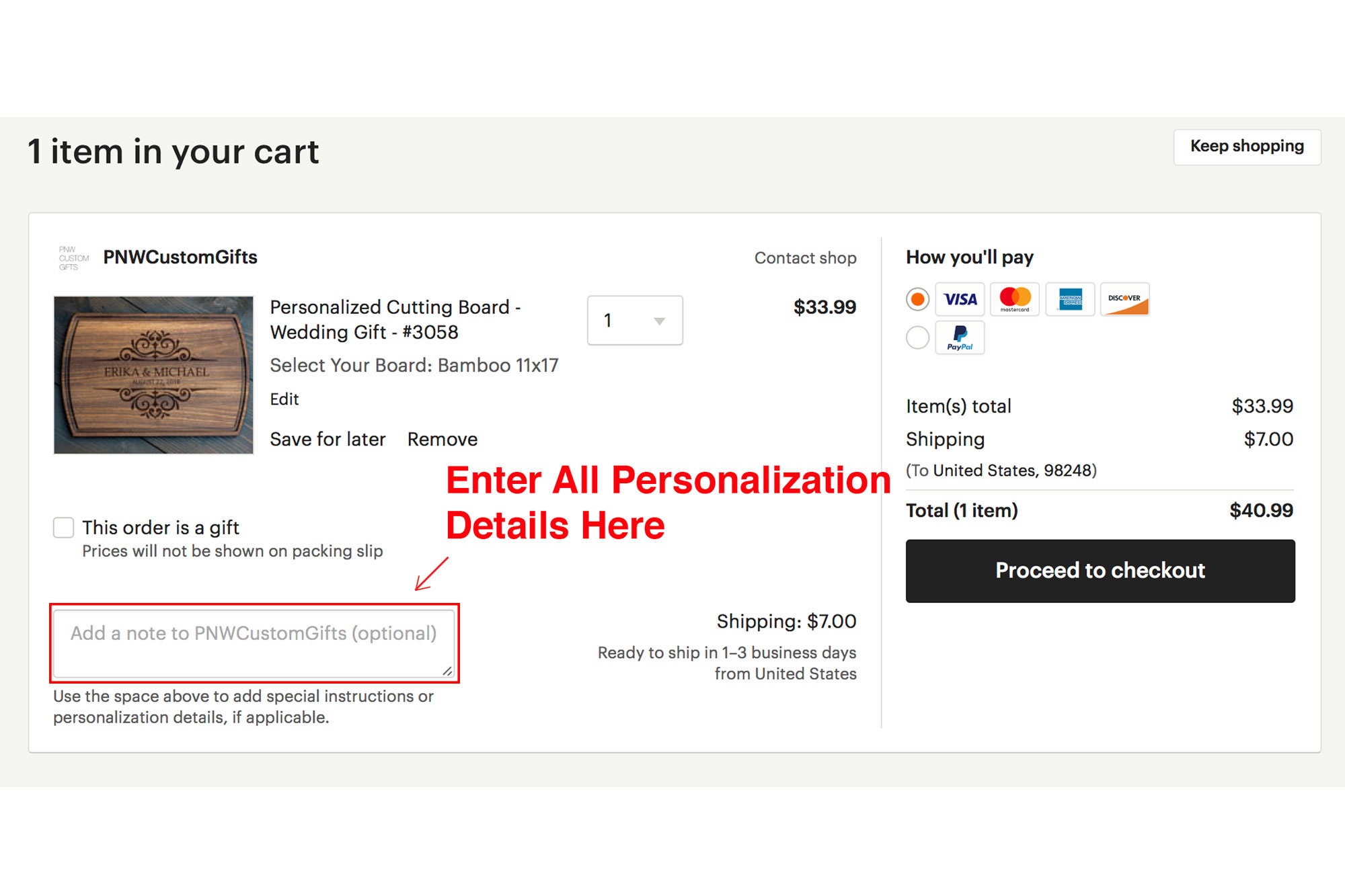A screenshot of an Etsy checkout page, featuring one item in the cart. The item, a personalized cutting board from the user "PNW Custom Gifts," is highlighted in black text at the top left, indicating "1 item in your cart." On the top right is a "Keep shopping" button for further browsing.

The cutting board, described specifically as a "Personalized Cutting Board Wedding Gift," is priced at $33.99. The buyer has selected an 11" x 17" bamboo board. The page also offers an option to add personalization, presumably for names or a special message, enhancing its appeal as a wedding gift.

Details about the order include a $7 shipping fee, with an expected shipping time between one to three business days. The total cost for the order amounts to $40.99. The layout and design elements closely resemble Etsy's interface, further confirming the platform.